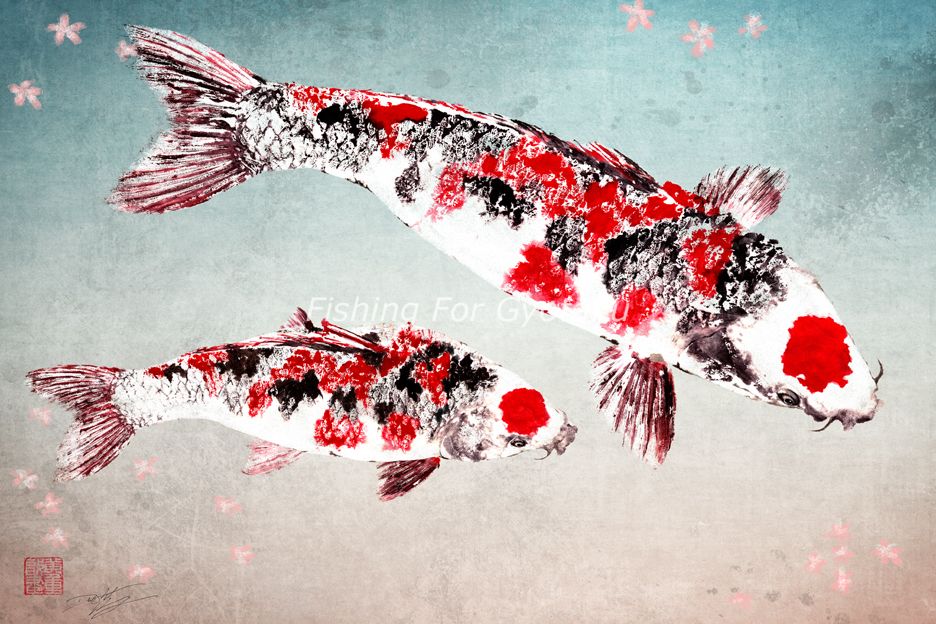This detailed painting showcases two koi fish against a gradient background that transitions from grayish blue at the top to dusty pink at the bottom, complete with small, five-petal pink flowers scattered throughout. Both fish exhibit a beautiful mix of white, black, and red coloration, with bold red circles on their foreheads and predominantly red, black, and white tails. The larger fish is positioned above the smaller one, and both have small whiskers and delicate front fins that resemble angel wings. The intricate patterns on their bodies further highlight the artistic style of the piece. In the center of the painting, faint white letters spell out "fishing for G.Y.O.," although the text fades into the fish and is somewhat difficult to discern. Adding to the authenticity and cultural essence of the artwork, a red stamp featuring Asian characters and a signature can be found in the lower left-hand corner. Additionally, there's a scannable emblem for more information located adjacent to the stamp.